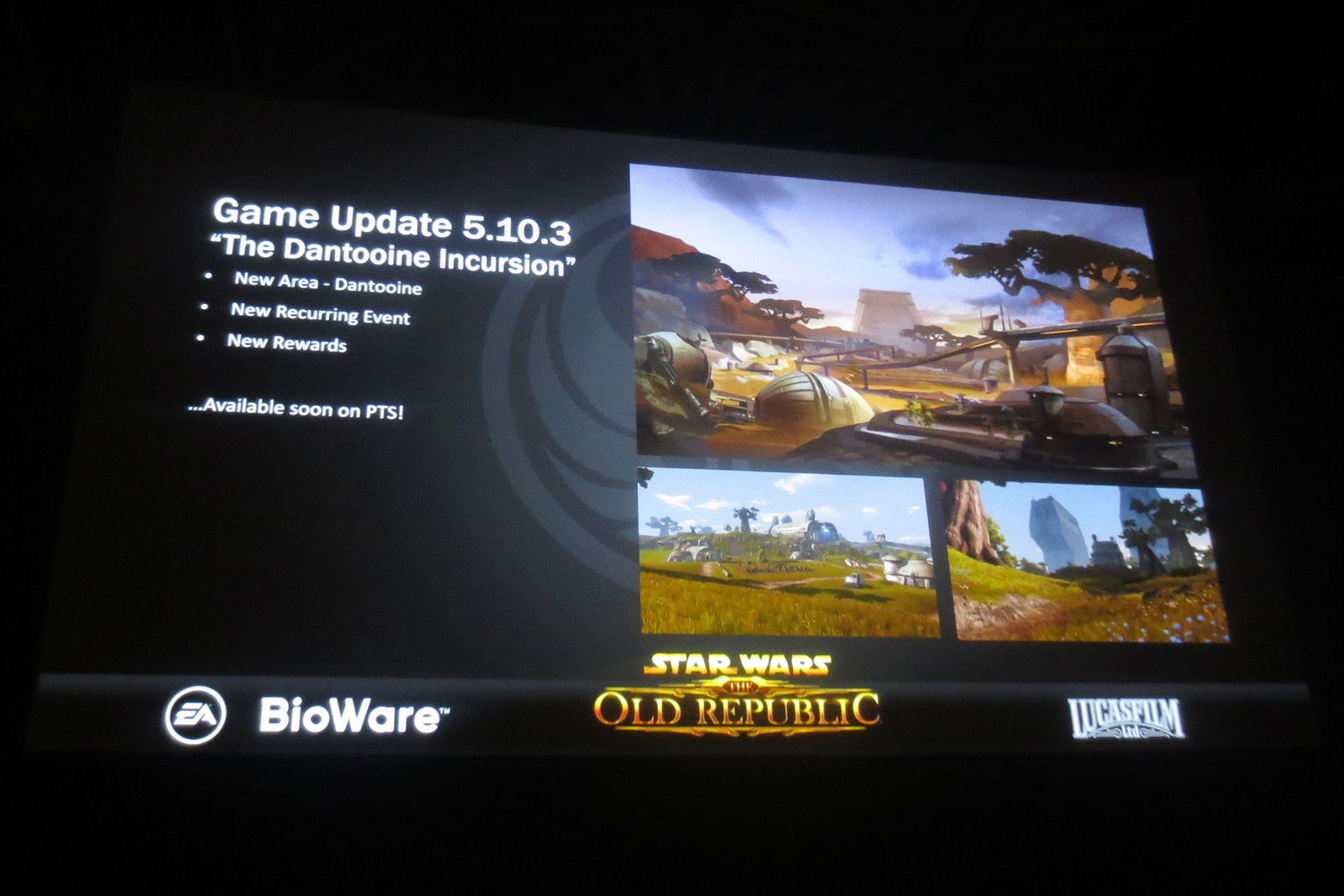The image is a detailed promotional still showcasing an upcoming update for a video game, displayed on a screen, likely from a movie theater or gaming setup. The upper part of the screen features a largely gray and white sky punctuated by hints of blue in an animated game screenshot. Dominating the right side is a massive tree with a round trunk and green leaves, beneath which sits a parked helicopter. Behind the tree stretches a rolling orange hill covered with more trees. Below this main image are two smaller pictures: the bottom left shows a large gray machine walking through a patch of mixed grass, interspersed with yellow grass, blue flowers, and yellow butterflies. The bottom right photo captures a green field populated with vehicles and trees, all under a sky filled with sizable clouds.

On the left side of the screen, against a black backdrop, white text announces "Game Update 5.10.3, The Dantooine Incursion." Three bullet points list "New Area: Dantooine," "New Recurring Event," and "New Rewards," ending with "Available Soon on PTS." At the very bottom of this promotional image, logos for EA and BioWare appear in a circle, and the text "Star Wars: The Old Republic" is flanked by the gold BioWare logo and the white Lucasfilm Limited logo.